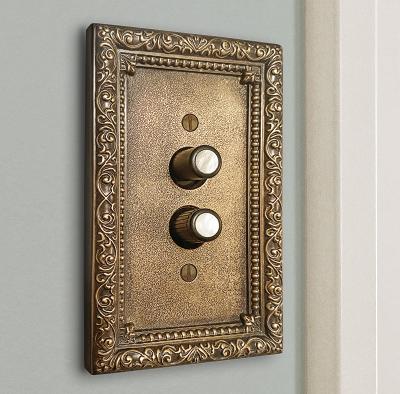This image is a detailed close-up of an antique-looking switch plate mounted on a light bluish-gray wall. The switch plate, which could be brass or bronze, features intricate, ornate edging and has a well-worn, vintage appearance. The plate is rectangular with a highly decorative design and is affixed to the wall with two darker brass screws located at the top and bottom. 

Centrally positioned on the plate are two circular knobs or dials, one above the other, which are likely for controlling the light or volume. These knobs are metallic with white centers and have perforations around their edges, suggesting they can be turned. Beside the switch, on the right side of the image, the edge of a white door frame is visible, further adding to the scene’s depth. The wall’s color is a light shade of blue-gray, complementing the ornate, metallic switch plate.